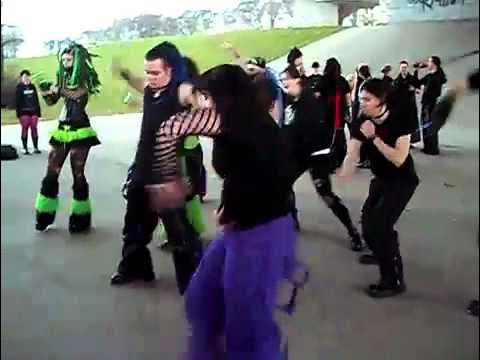In this detailed image, a large group of young people are gathered beneath an overpass, engaged in lively cyber goth dancing. The scene is characterized by a mix of thick, dated clothing predominantly in black, with some individuals standing out in vibrant colors. A woman in the foreground wears distinctive purple pants, fishnet sleeves, and a black shirt, while a man behind her sports an entirely black outfit and a blue ponytail. Another notable figure is a woman on the left with striking neon green hair styled in dreadlocks, accompanied by a neon green skirt and matching black and green fuzzy boots. The group appears diverse, some members thrashing their arms in rhythmic motion and others conversing and drinking from a large, indeterminate bottle. The setting is urban, with a green hill visible in the background next to the cement underpass. The atmosphere suggests a cyber goth-themed gathering or party, capturing a moment of animated interaction and mid-2000s fashion.